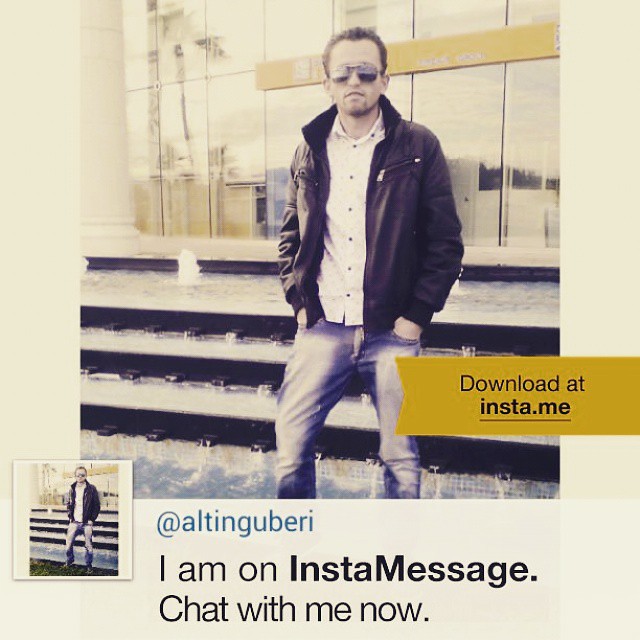A large square image features a man in his early 30s, with short dark hair and fair skin, standing confidently. He is dressed in a stylish black jacket over an unbuttoned white collared shirt, and he has both hands tucked into the pockets of his acid-wash blue denim jeans. Reflective black sunglasses shield his eyes, adding a hint of mystery. The man leans casually against dark stone steps that lead up to a glass-fronted building, which has bright, reflective floor-to-ceiling windows. A yellow sign with writing is prominently displayed across the front of the building. In the background, small waterfalls cascade gently downward, leading to a body of water. The scene suggests a mixture of urban and natural elements. 

Within the image, there is a yellow, underlined label on the bottom right that reads "download at insta.me" in black text. A smaller inset picture of the man is situated in the bottom left corner, adjacent to the blue text handle "@AltonGoobery." Below this, bolded text states, "I am on InstaMessage" with the invitation "chat with me now" in black print, indicating this is likely an advertisement for his presence or music on the platform.